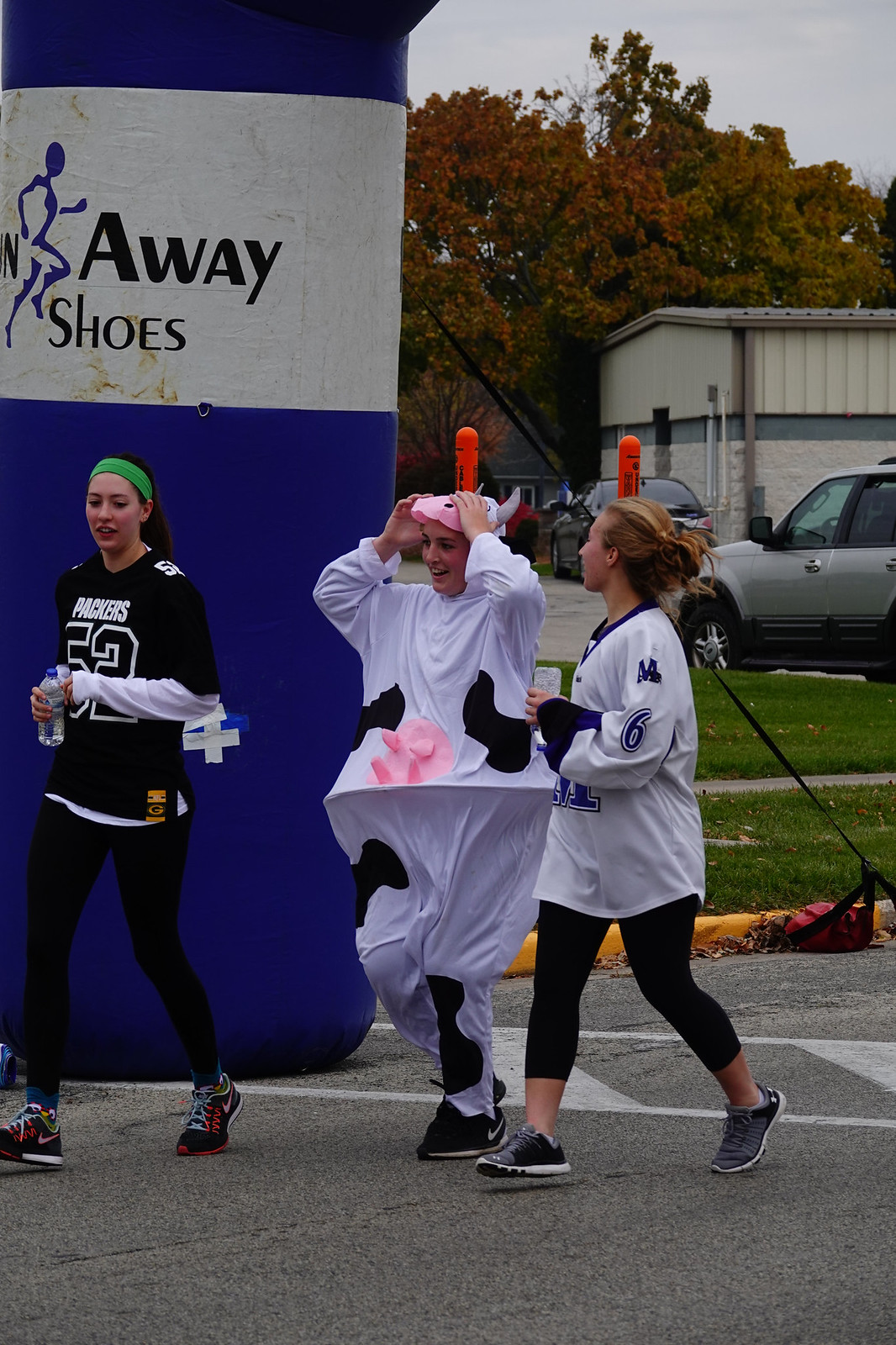In this tall rectangular outdoor photograph, three young women are running a race on a gray concrete surface marked with a white striped line. They are positioned left to right, making their way towards the left side of the image. The scene is set against the backdrop of a red and orange forest, adjacent to a gray building with a parking lot featuring several cars.

The leftmost runner is wearing a dark green Packers sweatshirt with the number 52 and an orange label at the bottom right. She pairs her outfit with a green headband, black leggings, and black sneakers, and carries a bottle of water in her hand.

The middle runner sports an eye-catching full-body cow costume, complete with black and white patches and fake red udders. She is smiling and has a hat decorated with cow horns. 

On the right, the third runner is dressed in a blue and white jersey with the number 6 and the letter M. She has blonde hair, blue sneakers, and black leggings that expose her ankles. She appears to be interacting with the middle runner.

Above the runners, there is a sign that reads "Something Away Shoes," and in the background are trees and an SUV building.